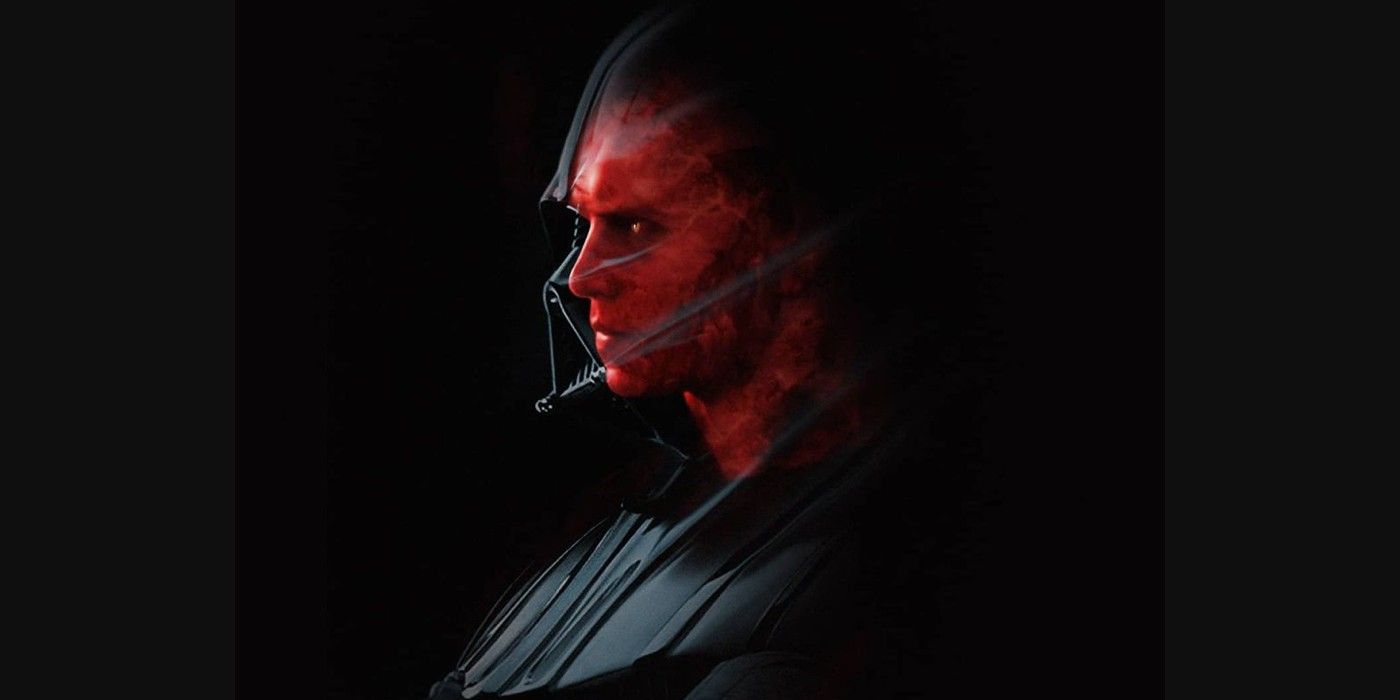The image is a highly stylized, heavily computer-generated or 3D-rendered portrayal of a villainous figure, reminiscent of Darth Vader from the Star Wars franchise. The central figure is encased in semi-transparent, reflective black armor, showcasing his shoulders and chest, with a distinct black helmet outlined against a stark, black background. This helmet features a prominent rebreathing mask with a large triangular vent where the mouth would be. Through the transparency of the helmet, the burnt, red, and charred features of Anakin Skywalker's face are visible, including his intensely glowing red eyes and smooth, hairless scalp. The villain is portrayed from the chest up, with a menacing gaze directed to the left. Flanking the central black square of the image are light gray borders on either side, suggesting that this could be a screenshot from a video, possibly concept art or a promotional image rather than a cinematic still. The image captures a moment post-transformation, highlighting the character's scorched visage beneath the iconic mask.